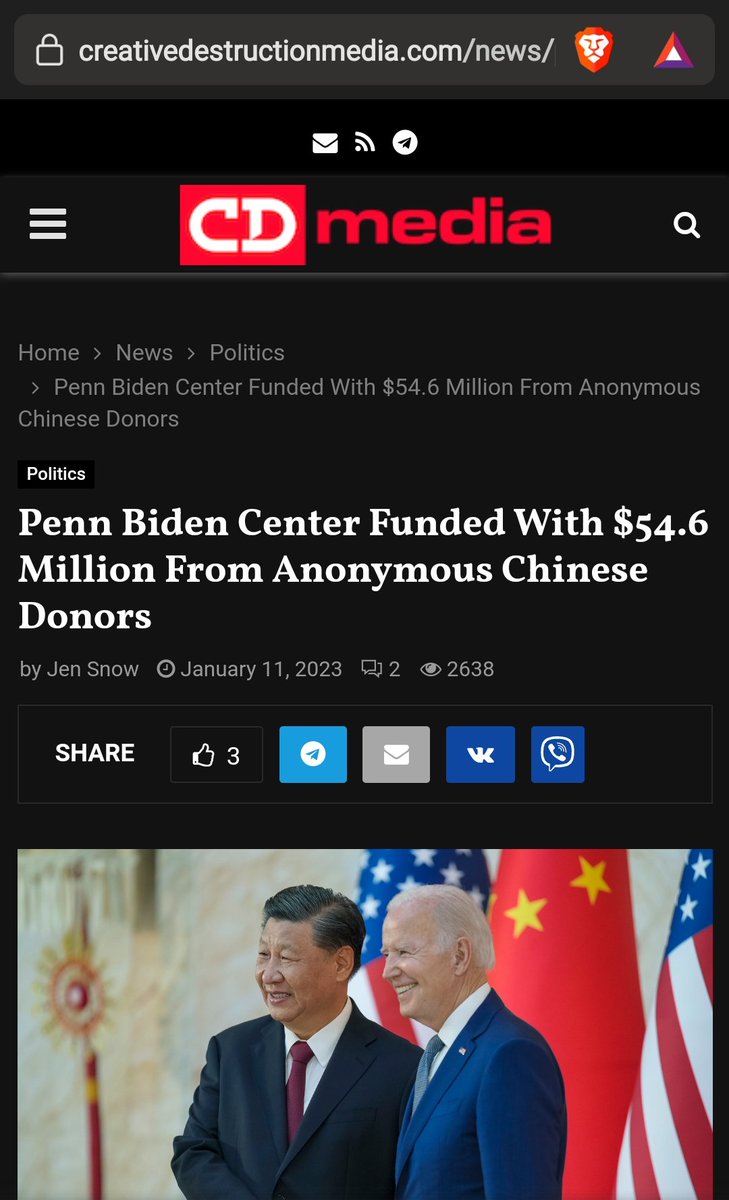**Cleaned-Up and Detailed Caption:**

The image displays a webpage from Creative Destruction Media featuring the headline, "Penn Biden Center Funded with $54.6 Million from Anonymous Chinese Donors." Authored by Jen Snow and published on January 11, 2023, the article includes social media sharing options and engagement metrics, indicating three likes and 2,638 votes. Beneath the article details, a photograph captures a moment of camaraderie between Chinese President Xi Jinping (left) and U.S. President Joe Biden (right), who are smiling and shaking hands. The backdrop prominently displays the flags of China and the United States, underscoring the international significance of their interaction.